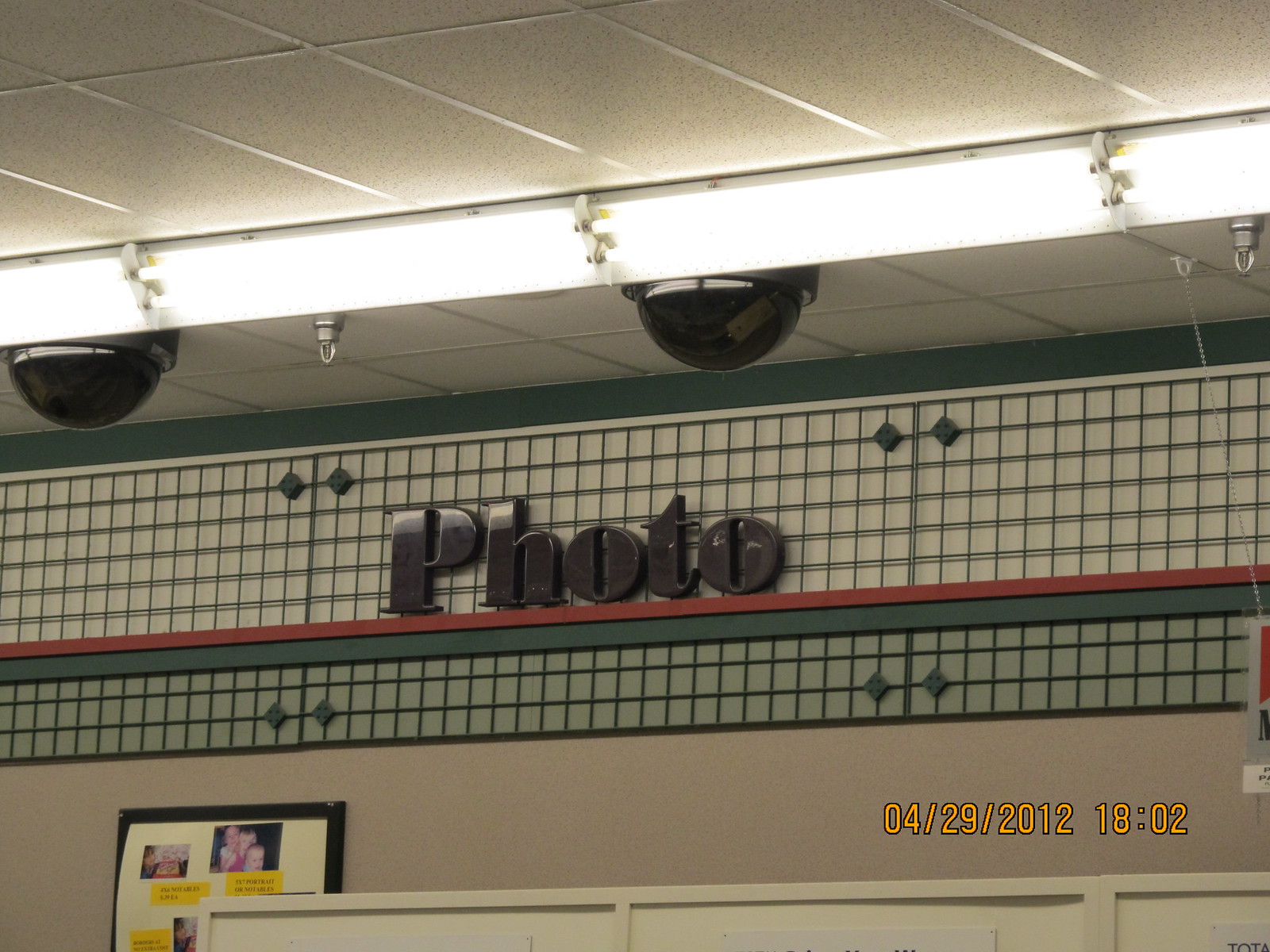The photograph captures the ceiling of a building with an intriguing mixture of elements. Dominating the upper wall is the word "PHOTO" emblazoned in large, textured black font that appears to be a tangible, three-dimensional installation rather than a flat print. The ceiling features several dome-shaped, black devices that resemble surveillance cameras, discreetly monitoring the area. Lighting fixtures are arranged in a pattern across the ceiling, providing illumination to the space.

The walls are a beige hue, adorned with a boxy pattern incorporating white, green, and interspersed with bands of red and green, creating a visually engaging backdrop. Near the bottom left-hand corner, a black-framed display stands out, showcasing photographs of children with yellow text beneath, adding a personal and lively touch to the environment.

In the bottom right-hand corner of the image, a timestamp reads "04/29/2012 18:02," anchoring the photograph with a specific date and time. This detailed and eclectic image blends architectural features with decorative elements to create an intriguing visual narrative.